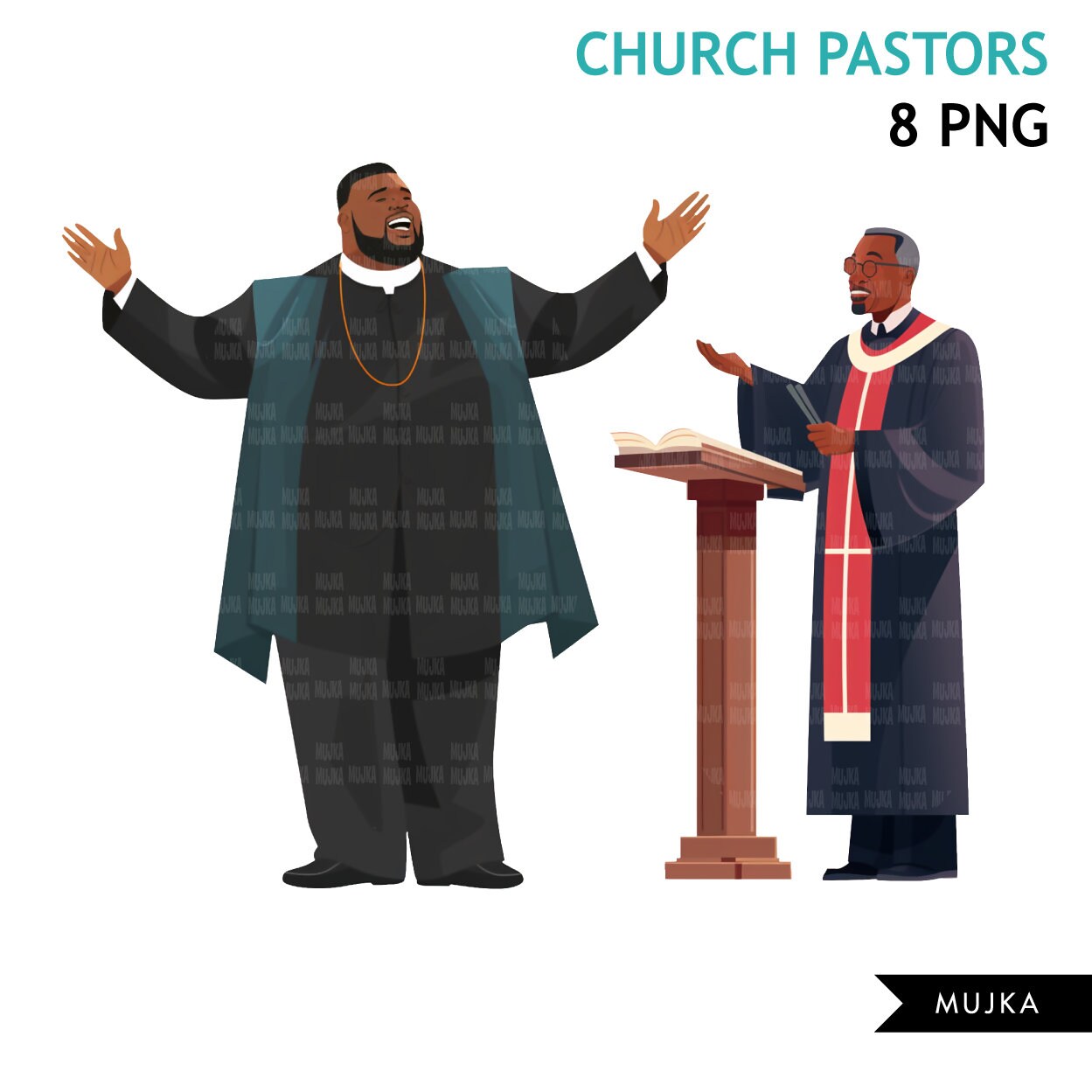The image showcases an animated drawing of two African-American church pastors, both engaged in religious activities. On the left, a large pastor with dark skin stands with his hands raised, appearing to preach or sing. He is dressed in a black suit with a blue vest and a white clerical collar, and he sports a gold necklace, black hair, and an O-shaped facial expression. On the right, an older, skinnier pastor stands behind a brown wooden pulpit with an open Bible. He wears a dark navy robe adorned with red and white accents, including a red sash with a white cross. This pastor has grayish hair, glasses, and extends his right hand in front of him, possibly delivering a sermon. The top right corner of the image features the text "Church Pastors" in blue and "8 PNG" in black. The bottom of the image contains a watermark with the name "Mujka," spelled M-U-J-K-A, in white text against a black background.